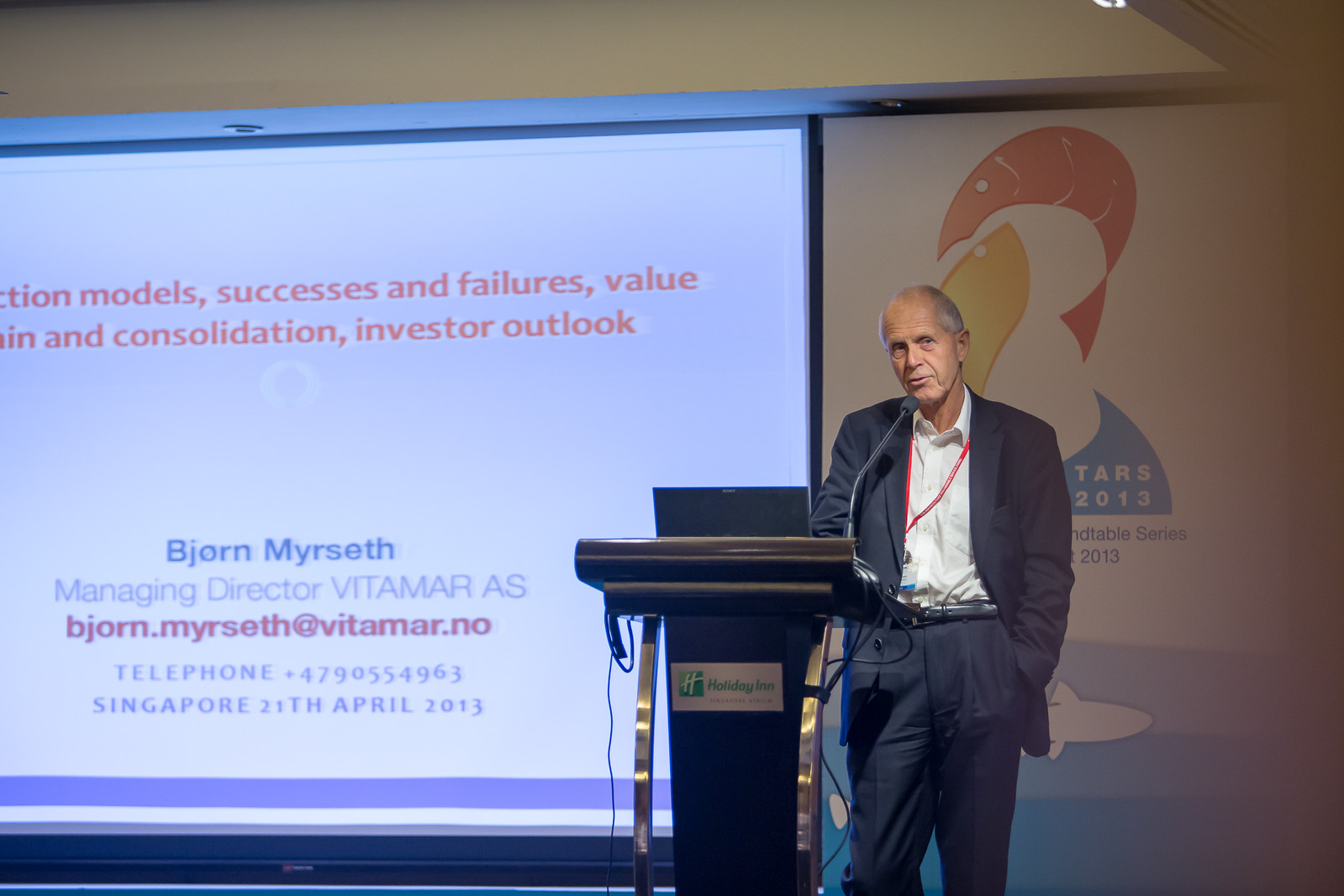The image depicts a man with short gray hair standing slightly to the right of a black podium on a stage. He is wearing a dark suit, a white button-down shirt, and a red lanyard around his neck, speaking into a microphone mounted on the podium. The podium features metal poles and a laptop or screen, along with a white "Holiday Inn" sticker.

Behind him to the left, a large projection screen displays fragmented phrases in pink text, including "action models," "successes and failures," "value," "consolidation," and "investor outlook." Below these, it identifies the speaker as Bjorn Meerseth, Managing Director of Vitamar AS, complete with contact information and the date, "Singapore, 20th April, 2013." To his right, there is a dimly lit screen with what appears to be an artistic image of a shark. The man is facing forward, slightly to the left, as he addresses his audience.